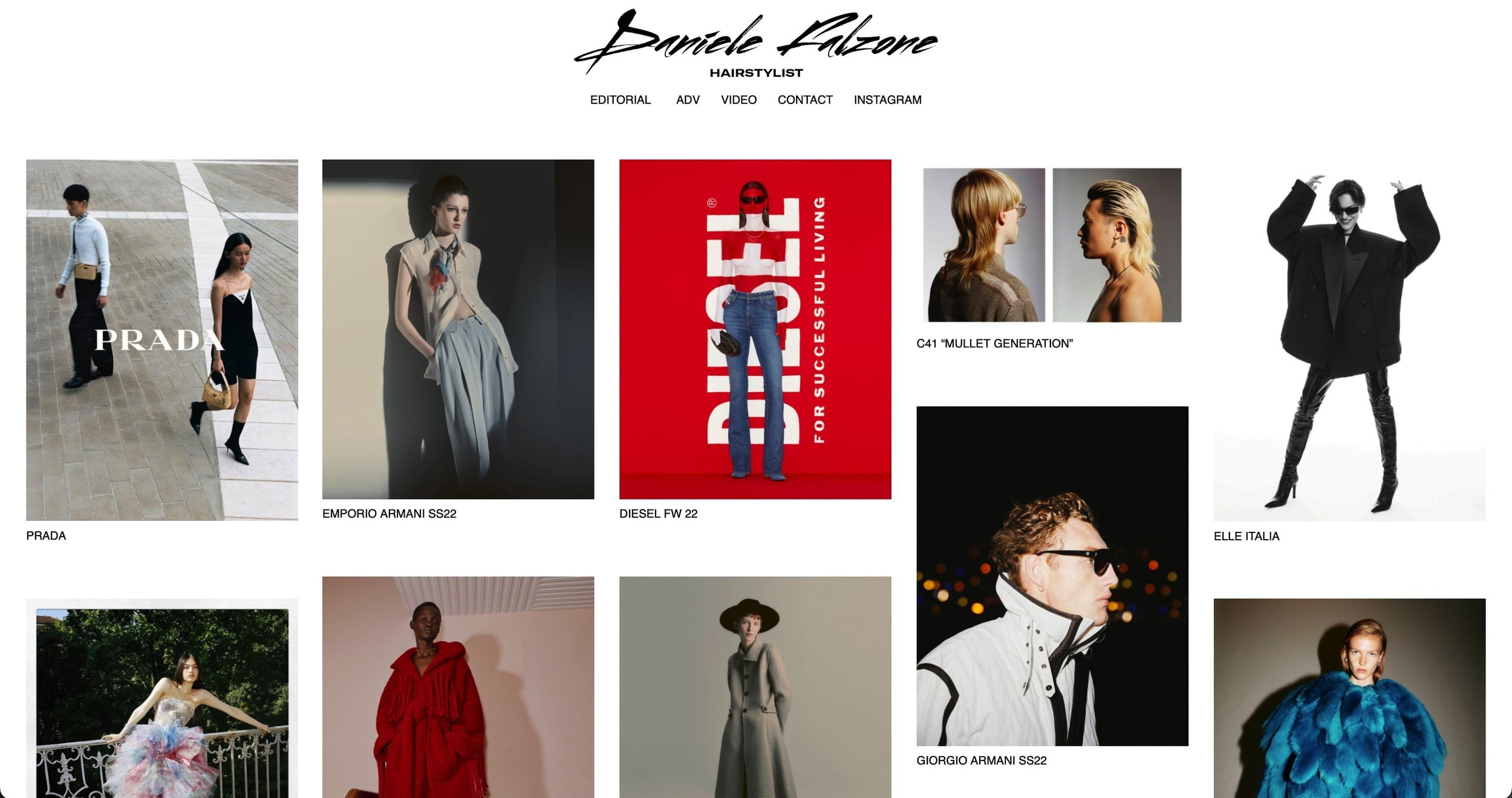This is a screenshot of a stylist's professional website. At the top, the name "Danielle Calzone" is prominently displayed in a stylized script, directly followed by the title "Hair Stylist." Below the title, there are five navigational links or buttons labeled "Editorial," "ADV," "Video," "Contact," and "Instagram." These buttons are neatly arranged for easy access.

Beneath the navigation bar, the page features a grid layout consisting of two rows filled with vibrant images of models and photographs. The first row showcases the following projects: "Prada," "Emporio Armani," "SS22," "Diesel FW22," "C41 Mullet Generation," and "L'Italia." Each image encapsulates Danielle Calzone's creative work, highlighting her expertise in styling for high fashion and editorial shoots.